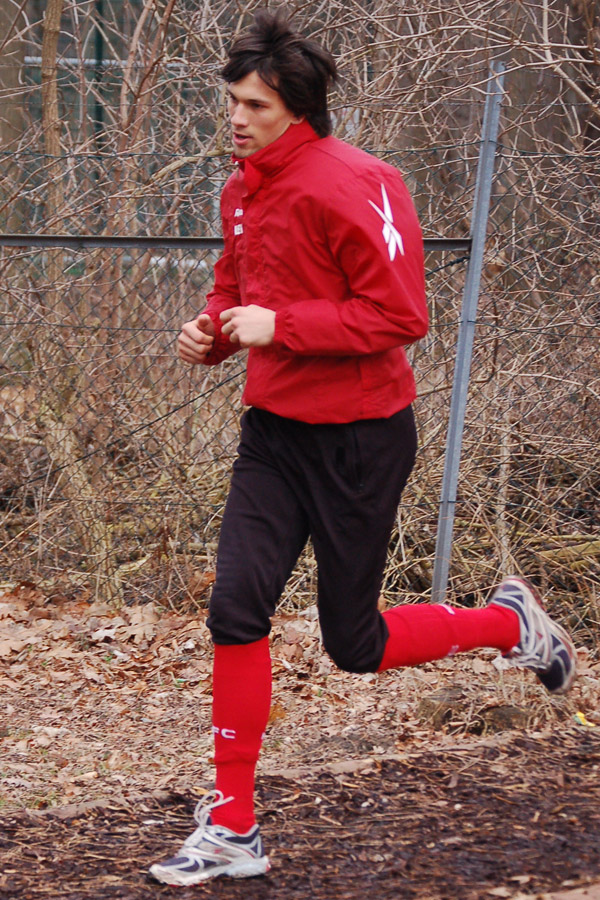In this detailed image, a young man with longish, dark brown to black hair jogs along a dark, well-trodden trail, seemingly made of black dirt. He is clean-shaven and dressed in a red athletic jacket adorned with a white Reebok emblem on the sleeve, paired with black jogging pants. Bright red socks extend up to just below his knees, complementing his white, blue, and red athletic shoes. His arms are positioned mid-stride, adding to the dynamic feel of his movement. The backdrop reveals a stark, late autumn or winter landscape, with dead, leafless trees and brown shrubbery. Dead leaves are scattered across the trail, and a dull gray metal chain-link fence runs alongside him. The overcast ambiance and the barren plant life emphasize the chilliness of the season. Additionally, in the distance, a soccer net is faintly visible through the lacework of the dormant branches.